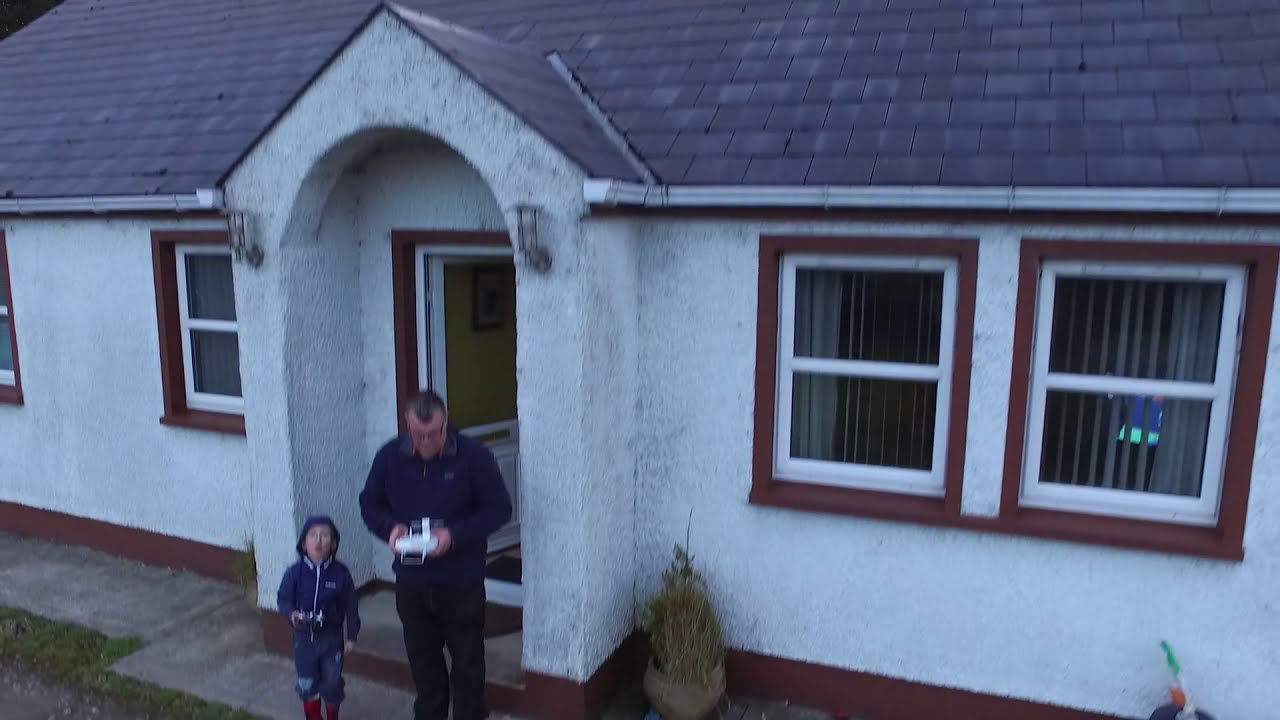In this photograph, we see an older man and a small child, about five years old, standing on the porch in front of the door to their house. The house is white stucco with an arched doorway and a gray or black shake roof, featuring dark windowsills and four brown-paned windows. The child, positioned to the left, is wearing a blue jacket with the hood up, complementing his blue pants and red boots or socks. He has a blue baseball cap and is looking up at the sky, holding a remote control, possibly operating a toy airplane or drone. The man, standing to the right, wears a blue coat, black pants, and glasses, and he holds a white and black object that also seems like a remote control. It appears to be drizzling outside. The photograph itself seems to be taken from a slight elevation, likely by the drone, as indicated by the angles and the reflection of a television visible through one of the windows.